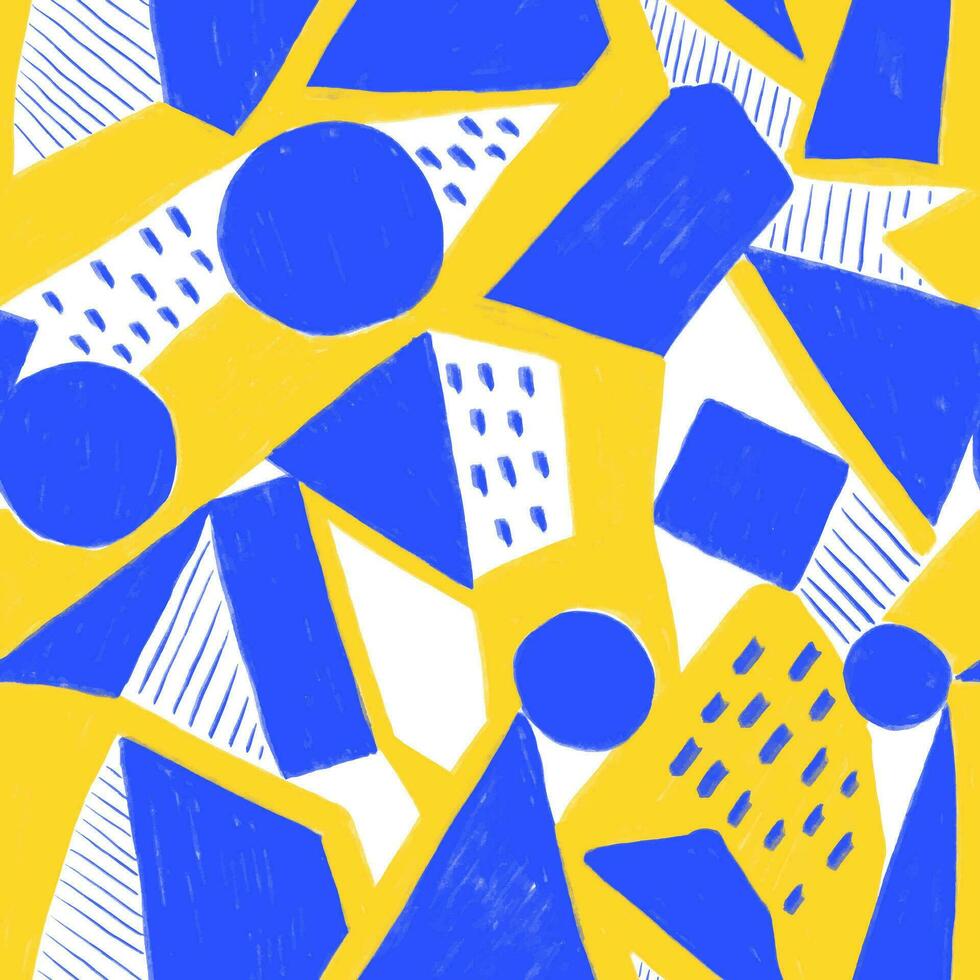This is an abstract painting on a paper canvas featuring a vibrant interplay of colors and shapes. The composition is dominated by three consistent colors: bright yellow, deep blue, and white. The white background is punctuated by a variety of shapes, including circles, squares, rectangles, and triangles, each intricately outlined with yellow brushstrokes. 

Four blue circles of varying sizes are spread throughout the painting, creating a dynamic vertical flow from the left to the right side of the image. Triangles with detailed vertical blue and white lines extend downwards, while other triangles adorned with blue dots punctuate the upper right corner. A dark blue square contrasts starkly against the white background in the center-right portion of the canvas.

Some shapes are described as having a texture or pattern reminiscent of a cheese grater, with blue stripes and dots adding to the visual complexity. Overall, the careful arrangement of shapes and colors against the white and occasional yellow background creates a vivid and engaging piece of abstract art.